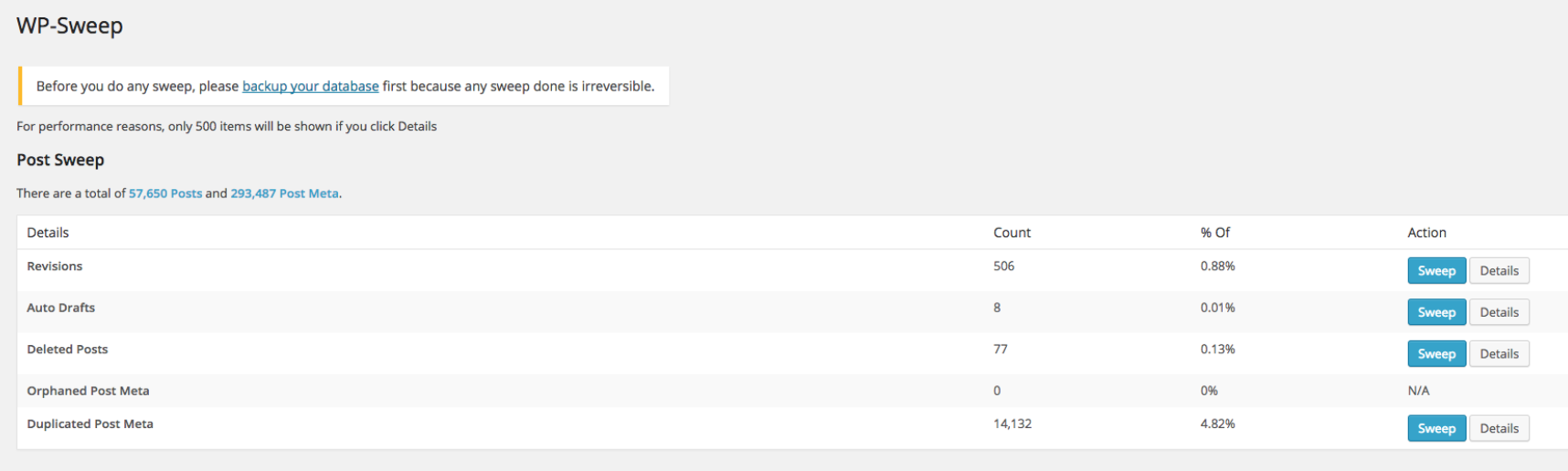Screenshot of a website displaying a detailed overview of a WordPress plugin named "WP Sweep." The header prominently says "WP Sweep," indicating that this tool provides insights into the user's post sweep activities. 

The main table is divided into three columns. The first column lists various categories related to posts, which include total posts (57,650), total post meta (293,487), revisions, auto-drafts, deleted posts, orphaned post meta, and duplicated post meta. Each of these categories represents different aspects of the website's content and metadata management. 

The second column displays the count for each corresponding category, showing how many instances exist for each type. There is also a percentage column, which likely indicates the proportion of each category relative to the total counts. 

The third column provides actionable options for each category, allowing the user to either initiate a cleaning action ("Sweep") or request more details ("Details") on the specific metadata. However, for the "Orphaned Post Meta" category, the action available in the last column is marked as "Not Applicable." 

This meticulously organized interface allows users to manage and optimize their WordPress database efficiently by removing unnecessary data, thereby enhancing website performance.